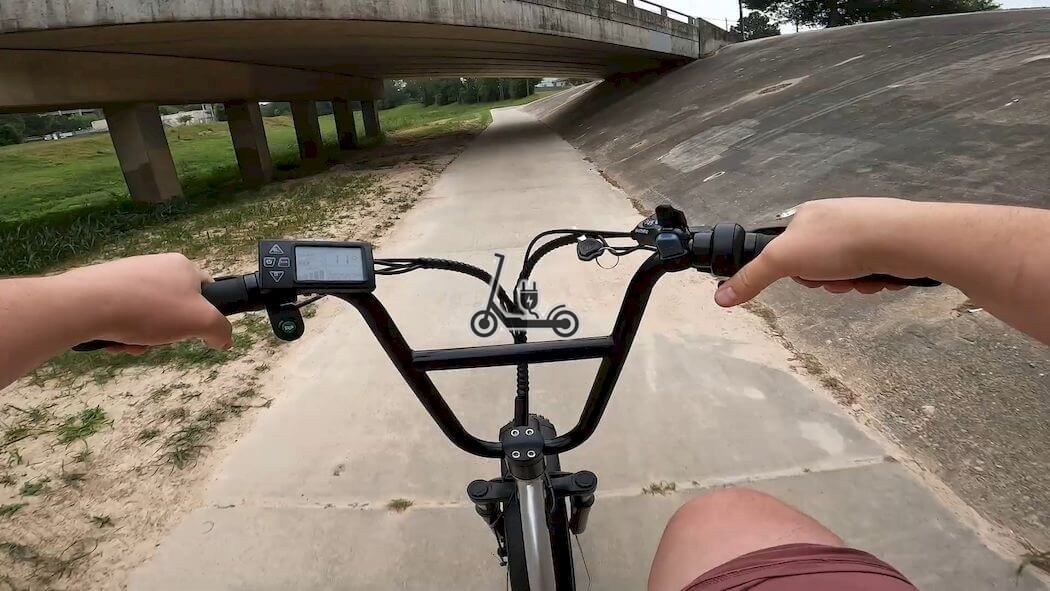A horizontally oriented photograph captures the dynamic perspective of a cyclist mid-ride. In the lower right quadrant of the image, the rider's right knee is partially visible. Both of the rider's hands can be seen gripping black V-shaped handlebars, complete with a central crossbar and a flat lower portion. A small gauge with a digital display is mounted at the end of the left handlebar, indicating possible speed or other metrics crucial for the ride.

An overlay icon featuring a long bicycle with tall handlebars and a plug with a lightning bolt further suggests this is an electric bike. The text and icon add contextual information, perhaps denoting battery levels or e-bike status.

The path ahead is a thin, pale gray cement walkway, bordered by a diagonal patch of asphalt on the right, which slopes down into the stone path. To the left, patches of dirt interspersed with sparse grass add texture to the landscape. 

The cyclist is approaching an underpass supported by five sturdy stone pillars, the bridge itself transitioning to a slate gray hue. Scattered sand partially covers the right edge of the path, spilling onto the cement. The scene provides a blend of natural and man-made elements, encapsulated under the looming structure of the bridge.